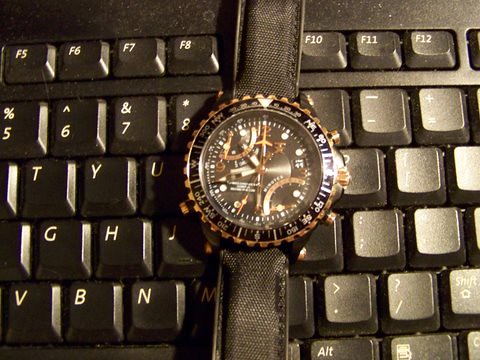In the image, a hand watch is prominently placed against a desktop keyboard, showcased in a vertical, close-up frame. The keyboard itself has thick, slightly protruding keys, and a variety of letters and symbols are visible, such as Y, H, G, T, commas, and semicolons. The watch is positioned in the center, with its black fabric strap extended both above and below the circular watch face. The watch's face is both a blend of old-school and modern aesthetics, with a gold jagged edge and a black inner ring. The dial features a clear section that reveals intricate, almost rusted brown gears, highlighting its vintage charm. Encircling the gears is a white ring marked with dashes indicating minutes and seconds, and an outer black border with numerical second markers. Completing the elegant design, a filigree-like border frames the watch, solidifying its classy appearance amidst the utilitarian backdrop of the keyboard.